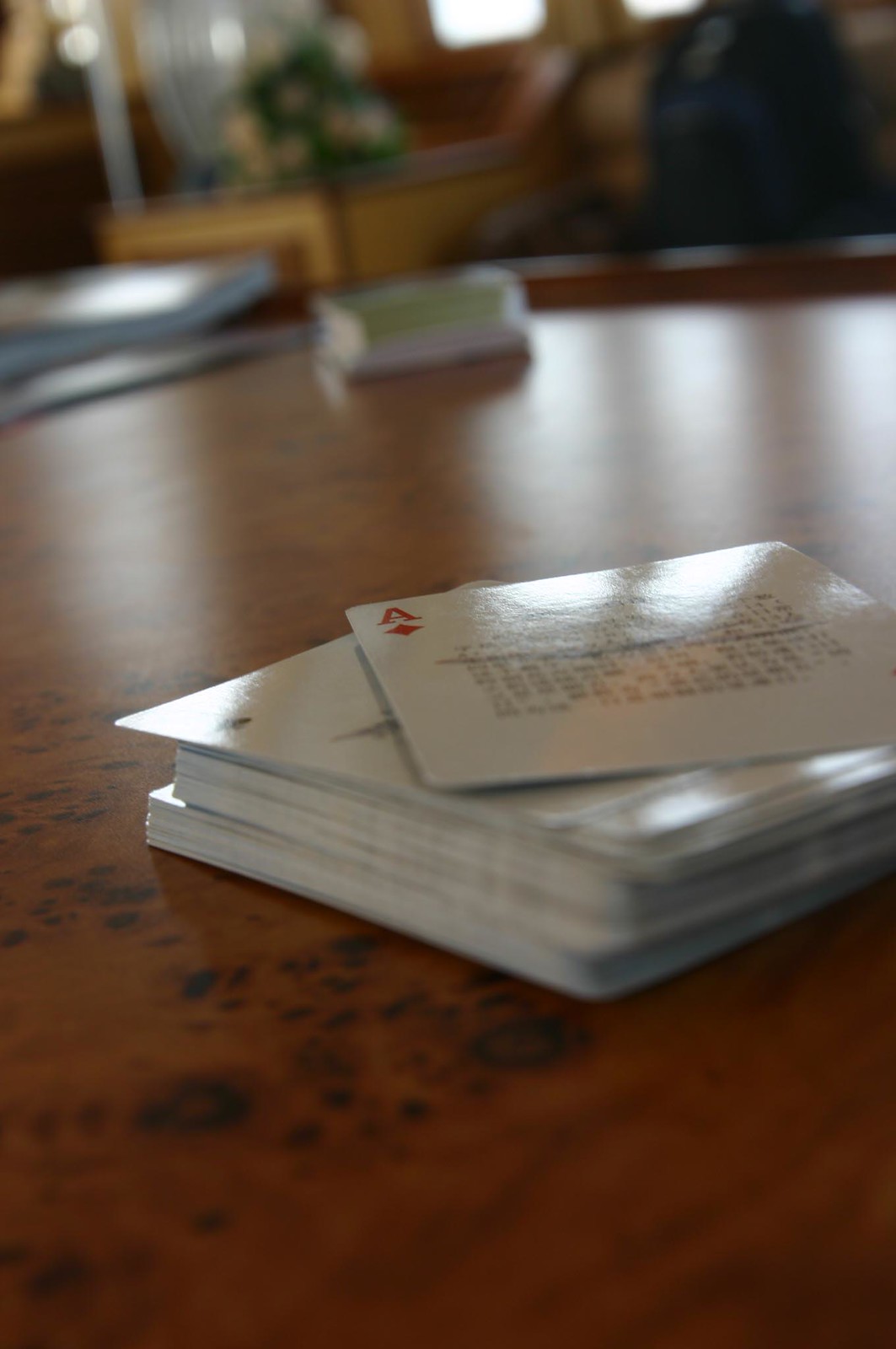This portrait-oriented photograph showcases an ultra-close-up view of a unique deck of playing cards. The image focuses primarily on the top card, an Ace of Diamonds, easily identifiable by the prominent 'A' and the diamond symbol. The cards have a strikingly glossy finish, with a white background and black text that appears to form an intricate pattern, though the exact design is blurred by the reflective surface, which catches the ambient light in the room. The deck is slightly fanned out, revealing only the edge of the next card beneath the Ace. These cards rest on a richly patterned, brown wooden table, the surface marred with dark, irregular blotches suggestive of an exotic wood. In the background, the blurred outline of another deck of cards is faintly visible, adding depth to the composition while keeping the primary focus on the glossy, enigmatic Ace of Diamonds. The room’s further details remain indistinct due to the pronounced bokeh effect.